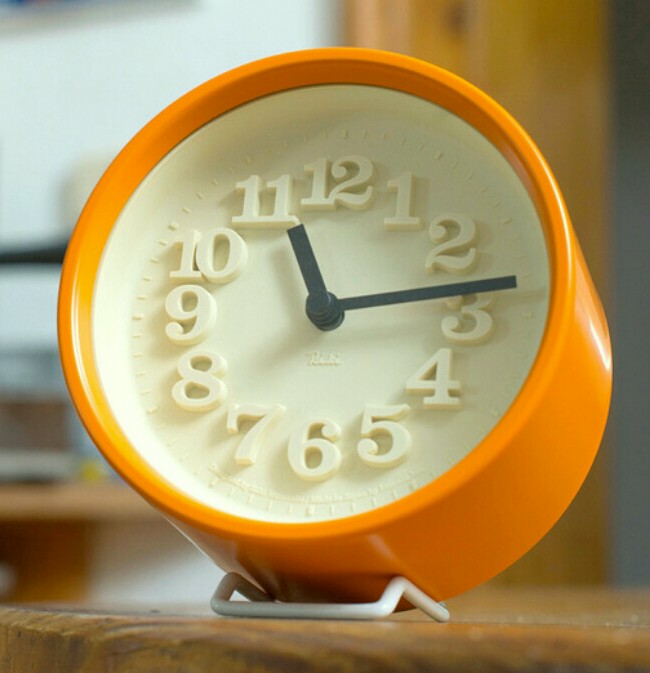This image showcases a charming, vintage clock reminiscent of the 1970s. The clock's all-plastic construction features a striking orange outer shell, contrasted by a cream or off-white clock face. The black minute and hour hands stand out prominently against the monochromatic background. The numerals, matching the clock face in color, are arrayed in a traditional circular fashion. The clock is slightly inclined, facilitated by a small wire stand integrated into its design. It rests on a wooden table, adding to its nostalgic appeal.